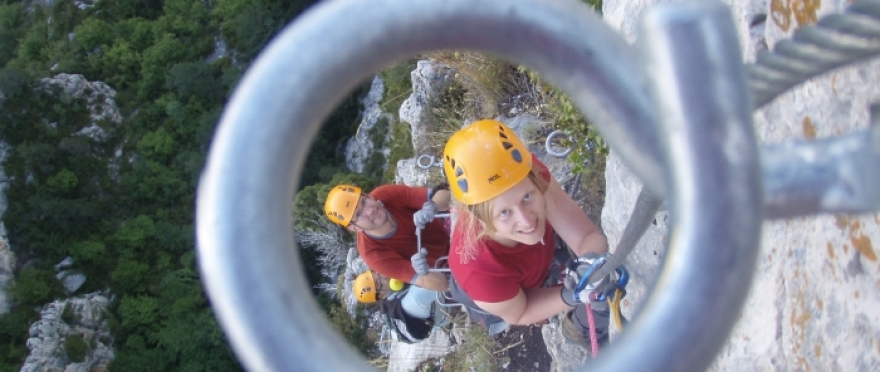In this unusual and striking image, we see a dramatic rock climbing scene captured from a unique vantage point. The photograph is taken looking through a close-up metal ring, likely part of the climbing equipment affixed to the rock face. Framing the climbers within the ring, the image provides a powerful perspective of the climb. 

In the center of the frame, we see three determined climbers scaling an actual mountainside, with hooks and ropes securely fastened into the rock. The foreground prominently features a woman with blonde hair, wearing a red t-shirt and yellow helmet, gripping a rope with gloved hands. Directly behind her, a young man in a red shirt and yellow helmet, possibly with glasses, is also holding the rope. Further back, a third climber wearing a grey t-shirt and backpack, and donning a yellow helmet, follows the ascent. 

The photo captures the steep and rugged terrain of the climb, with scattered rocks and patches of grass beneath them. Background details reveal a natural setting with trees and additional rock formations, emphasizing the height and challenging nature of this rock climbing expedition. This compelling image beautifully encapsulates the thrill and intensity of outdoor climbing adventures.